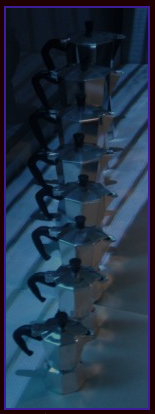The image displays a tall, narrow photograph featuring eight classic Italian coffee pots, arranged in a neat, ascending row from the bottom to the top of the image. Each pot, made of shiny metallic material with faceted sides and a flared stout base, reflects the light streaming in from the lower left to the upper right. The coffee pots have black handles and lids with black knobs, positioned such that the handles face left and the spouts face right. Sunlight or overhead lights cast long shadows and vertical stripes across the pots, creating a dynamic interplay of light and shade on the reflective surface and throughout the overall bluish-tinted composition.